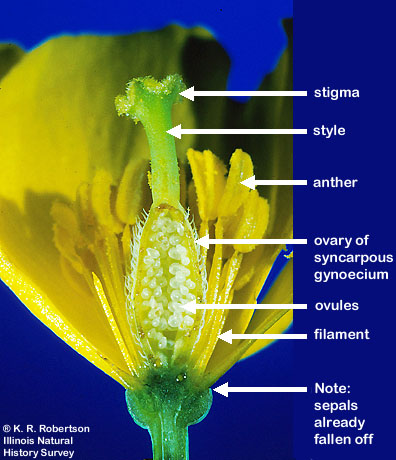The image is a detailed, vertical diagram of a yellow flower, set against a predominantly deep royal blue background. The diagram focuses on a labeled cross-section of a flower, with a side-by-side photographic and textual representation. 

On the right-hand side of the image, there is a darker blue vertical banner listing the flower parts in white text, along with arrows pointing to the corresponding sections of the flower. This text includes "Stigma" at the top, followed by "Style", "Anther", "Ovary of Syncarpous Gynosium", "Ovules", "Filament", and a note stating "Sepal has already fallen off."

The left side of the image displays the flower itself, showing the intricate internal structures. The flower is predominantly yellow, with some green in the middle section, and visible seed-like structures in the cutout part, highlighting the ovary and ovules. The petals are intact and spread out against the blue background, with the stem visible and cut in half to show its inner parts.

Additionally, in the lower left corner of the diagram, there is a copyright attribution, reading "K.R. Robertson Illinois Natural History Survey."

This comprehensive illustration effectively labels and points out each part of the flower, providing clear educational insight into its anatomy.